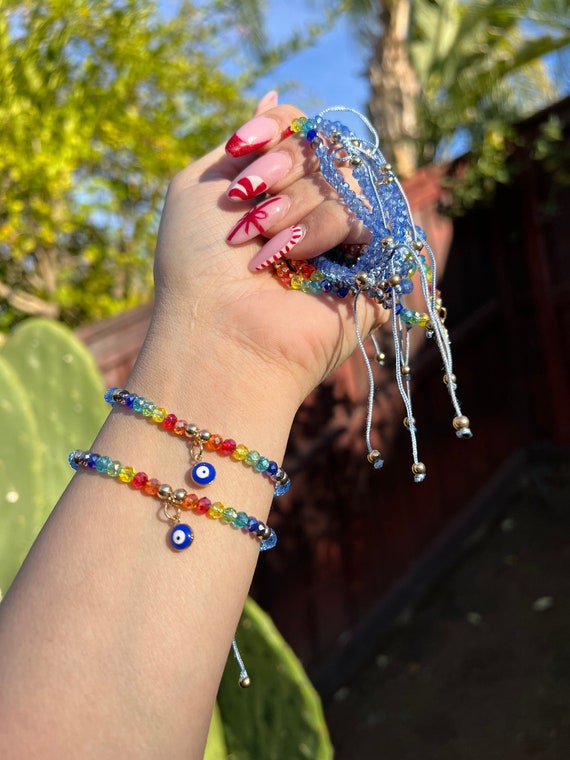A detailed color photo shows a close-up of a forearm and hand raised against a daylight sky. The rectangular image, taller than it is wide, captures the palm side of the hand, fingers closed. The fingernails are overly long, fake, with a pink background adorned in red and white peppermint-like designs; a red bow embellishes the ring finger's nail. Two rainbow-colored friendship bracelets, made of plastic beads in dark blue, light blue, clear, yellow, red, and orange, adorn the wrist. The bracelets feature small evil eye charms with blue borders hanging off them. The hand clutches additional bracelets, predominantly with translucent blue and rainbow beads, and a blue string with gold and blue beads dangles from them. Set outdoors under the sun, the vibrant background includes a large cactus, green leaves, trees, and a hint of a brick wall. There are elements like a red fence and possibly fairy-wing-like greenery adding charm to the setting. The bottom right-hand corner of the image is notably darker, nearly black.